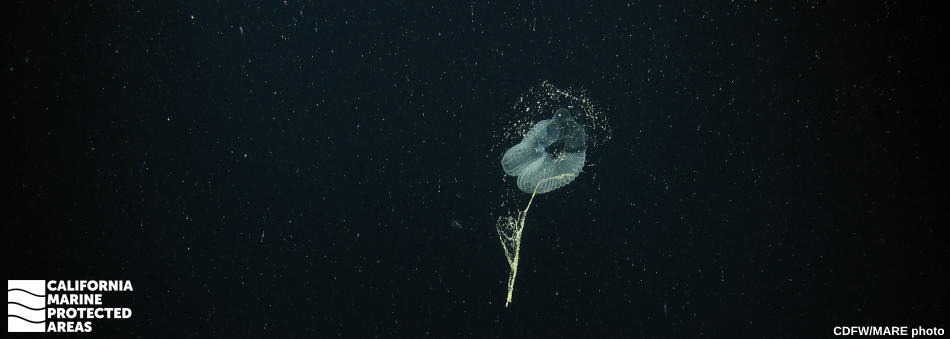This image captures a captivating photograph of a glowing, semi-transparent jellyfish-like marine creature floating in the dark depths of the ocean. The backdrop is a solid black, emphasizing the luminescent, bluish-green hues of the jellyfish at the center of the frame. Surrounding the jellyfish, there are tiny particles and bits of debris, reminiscent of underwater pollen, imbuing the scene with an ethereal quality. The photograph, which seems either taken underwater or possibly magnified, also features two key annotations: in the bottom left corner, a white logo reading "California Marine Protected Areas," and in the bottom right corner, the white text "CDFW MARE Photo." The overall composition of the image is a very long rectangle, accentuating the depth and mysterious beauty of this underwater spectacle.